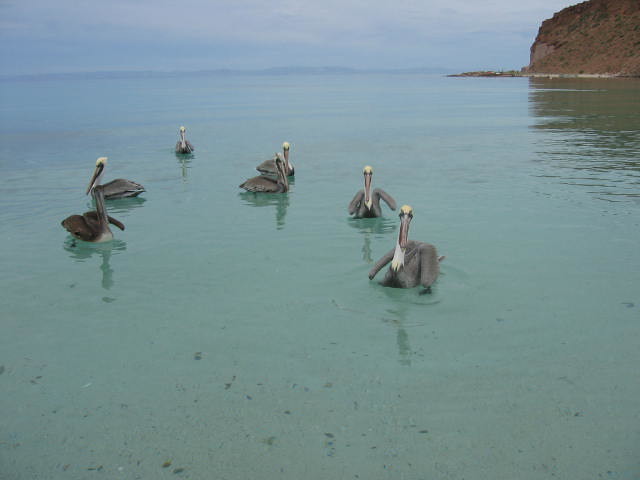The photograph showcases a serene natural setting featuring a cluster of approximately six to seven birds wading in a calm, bluish-green body of water. The water is fairly clear but not crystal clear, giving it a slightly murky appearance. The birds, identified as cranes or possibly pelicans, exhibit a brownish-gray coloration with white necks and heads, featuring long, skinny beaks with hints of white towards their tips. Among the group, three birds face the camera, one crane turns its neck backward, while another faces to the left.

Dominating the background are cloudy skies with glimpses of a distant, blurry horizon line where the water meets the sky. To the right, a significant land formation, described as a brown cliff or rocky outcrop, adds to the scenic beauty. The birds, appearing to enjoy their tranquil environment, are positioned centrally and slightly to the left within the composition.